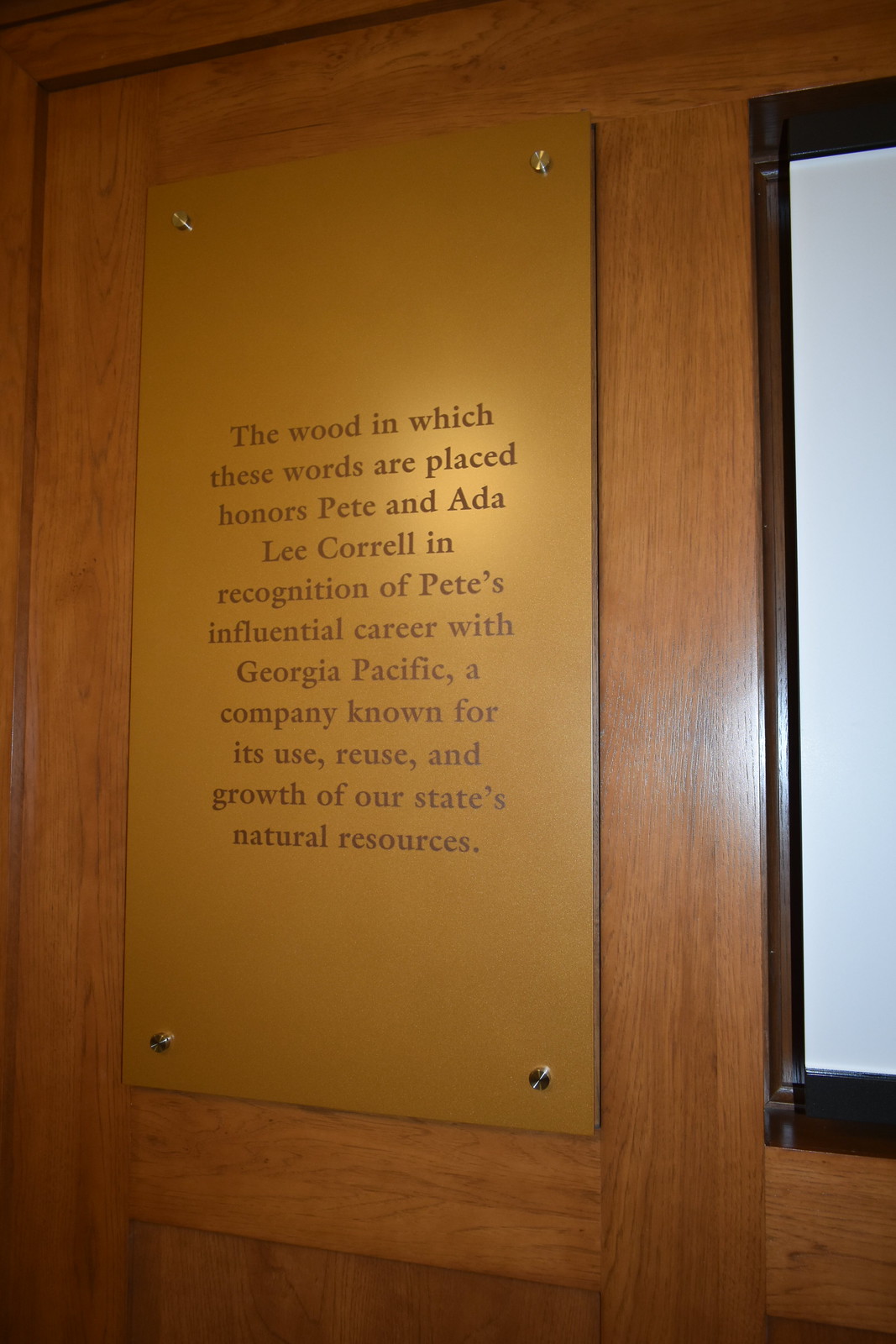The image portrays a highly ornate and polished wooden wall, possibly made of maple, featuring detailed woodwork reminiscent of an elegant office setting. Prominently displayed on the wall is a gold-colored, brass plaque, secured with four silver screws at each corner. The inscription on the plaque reads, "The wood in which these words are placed honors Pete and Ada Lee Correll in recognition of Pete's influential career with Georgia Pacific, a company known for its use, reuse, and growth of our state's natural resources." Adjacent to the plaque, on the right-hand side, is a rectangular section containing what appears to be a glass panel, framed in black, with a white background, which could be part of a door or a framed picture. The image appears to be zoomed in, showing only the top portion of this detailed wall and its elements.